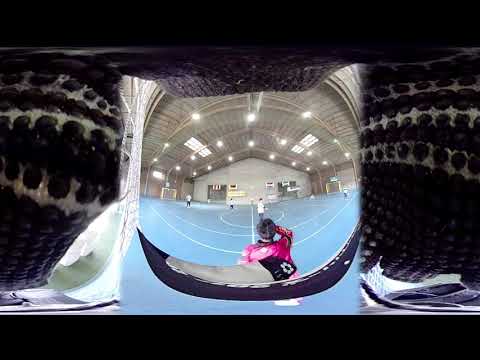This color photograph captures an indoor soccer game set within a sports arena featuring a concrete building with a large metal roof equipped with both electric lights and skylights. The blue playing field with distinct white lines is at the center of this photograph, with goals visible at each end. The image appears to be taken with a fish-eye lens, giving it a circular, distorted view. Standing prominently in the foreground is a person wearing a pink shirt with black stripes and a black hat, facing away from the camera with one arm raised to their head. Scattered around the field are other players, emphasizing the ongoing game. The image is framed by black bars at the top and bottom, indicative of a still captured from a video. Additionally, parts of the image are overlaid with a black and white reptile-skin-like pattern, creating an impression that the photo has been photoshopped or superimposed onto another background.